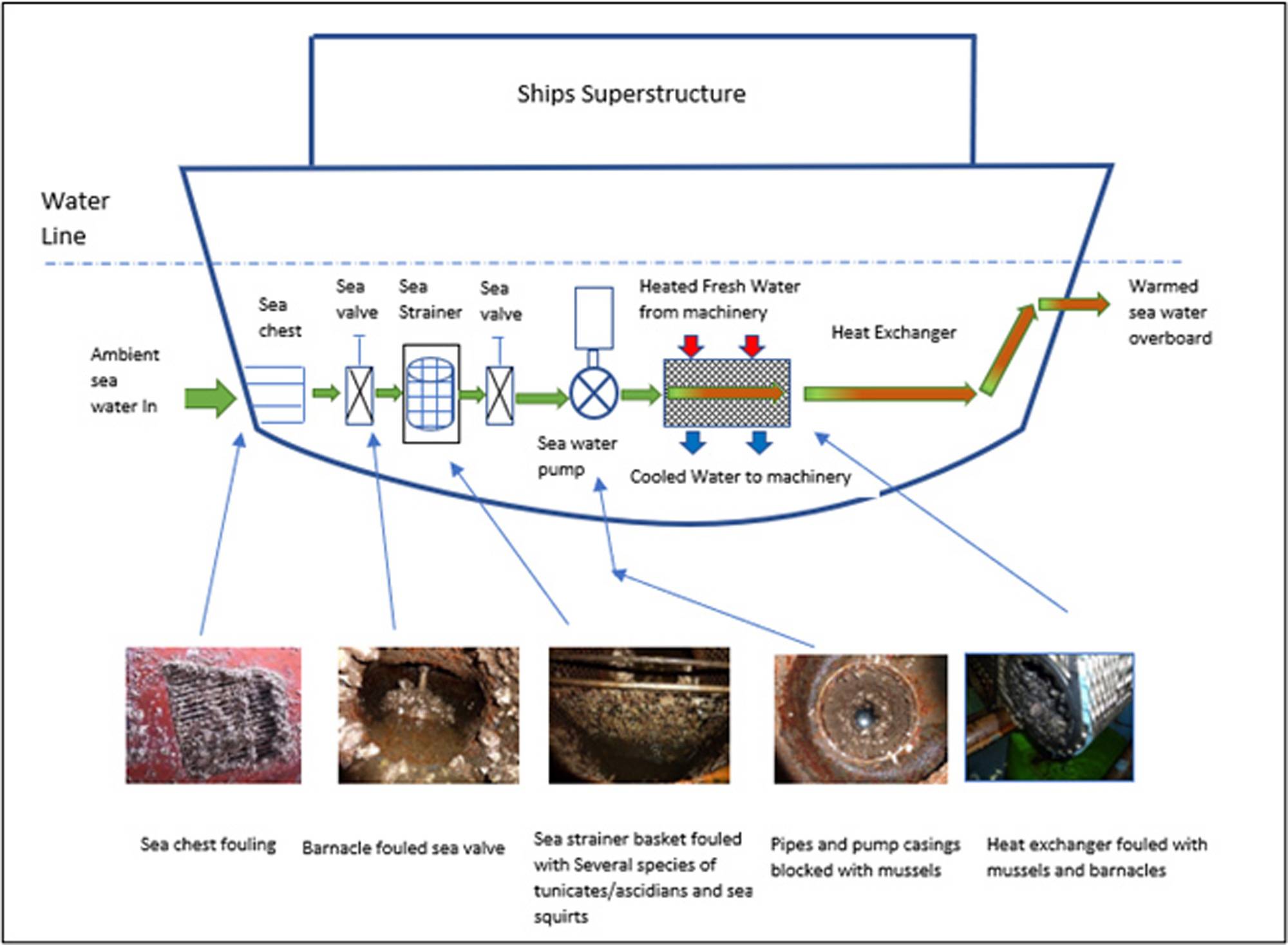A detailed sketch of a ship's superstructure illustrating a water purification system, with intricate depictions of potential marine fouling points. The upper part of the diagram represents the ship's outline, denoted with "ship's superstructure," and features a dashed line marking the waterline. Below this line, the diagram becomes highly detailed, showcasing the flow of ambient seawater through various stages inside the ship. Water enters through a section labeled "ambient seawater in," proceeding to the sea chest, sea valve (illustrated as a square with an X), and sea strainer (depicted as a cylindrical grid pattern inside a rectangle). Next, it flows through another sea valve, a seawater pump (a series of rectangles and circles), and heated freshwater from machinery (with red and blue arrows indicating temperature changes in a grid-patterned box). The final components include a heat exchanger (with gradient color arrows) and the exit point marked "warmed seawater overboard."

Below the main schematic, there are small photographs illustrating real instances of fouling, pointing to their respective components in the diagram: a sea chest fouled with marine life, a barnacle-coated sea valve, a sea strainer basket clogged with various species, pipes and pump casings blocked by mussels, and a heat exchanger fouled with mussels and barnacles. The text annotations throughout the diagram are rendered in a basic sans serif font, providing a clear and concise understanding of the flow and potential problem zones within the ship’s water purification system.